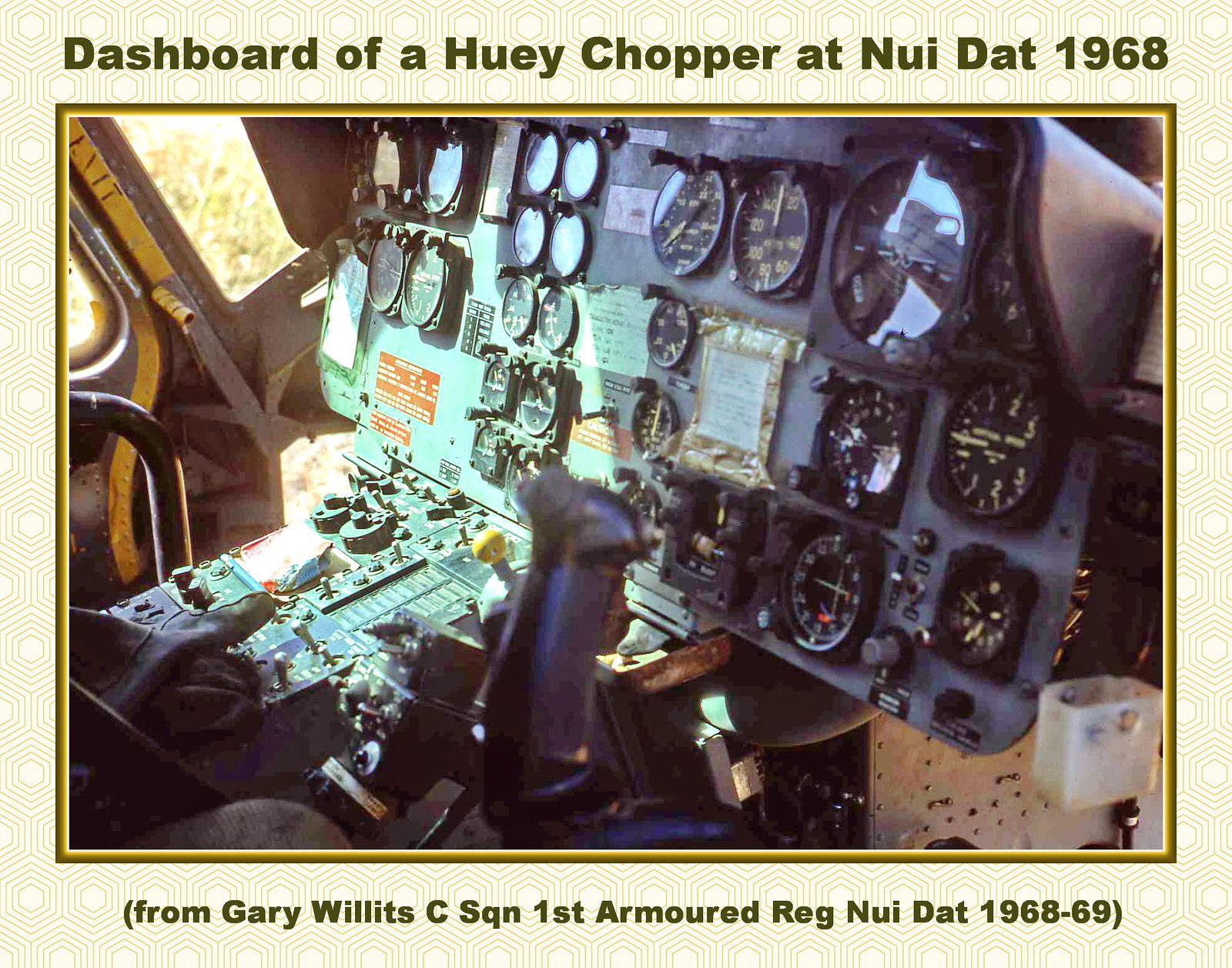The image depicts a horizontally aligned, vintage color photograph of the dashboard inside a Huey chopper at Nui Dat from 1968. The photograph, framed within a hexagonal pattern border outlined in brown and gold, features detailed, realistic visuals of numerous circular gauges and measurement devices, all predominantly in black. The dashboard is angled, appearing larger on the right side, with a small section of the helicopter window visible on the top left, offering a glimpse of the outside. Above the image, the headline in olive green or black text reads, "Dashboard of a Huey Chopper at Nui Dat, 1968." Below, a subhead in matching text states, "(from Gary Willis, CSQN, First Armored Reg, Nui Dat, 1968-69)."